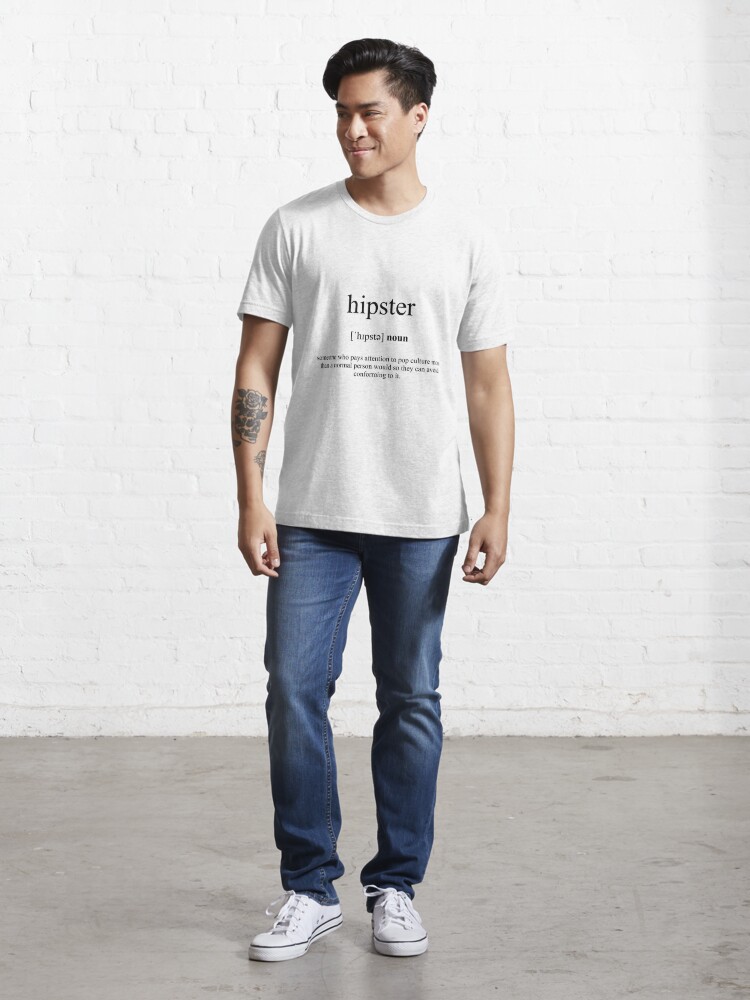In this image, we see an Asian man with medium brown skin, short dark hair that's longer on top, and neatly styled. He appears to be modeling clothes, standing confidently in a warehouse setting with a gray concrete floor that shows a slight reflection and a rough, painted white brick wall behind him. He is dressed in a white graphic t-shirt which features the word "hipster" in large black letters, followed by the phonetic spelling "noun" and a definition below in smaller black text around the middle of the shirt. He completes his outfit with dark blue denim jeans and white sneakers. The man is smiling and looking off to his right, showcasing a tattoo of a rose and skull on his right forearm.